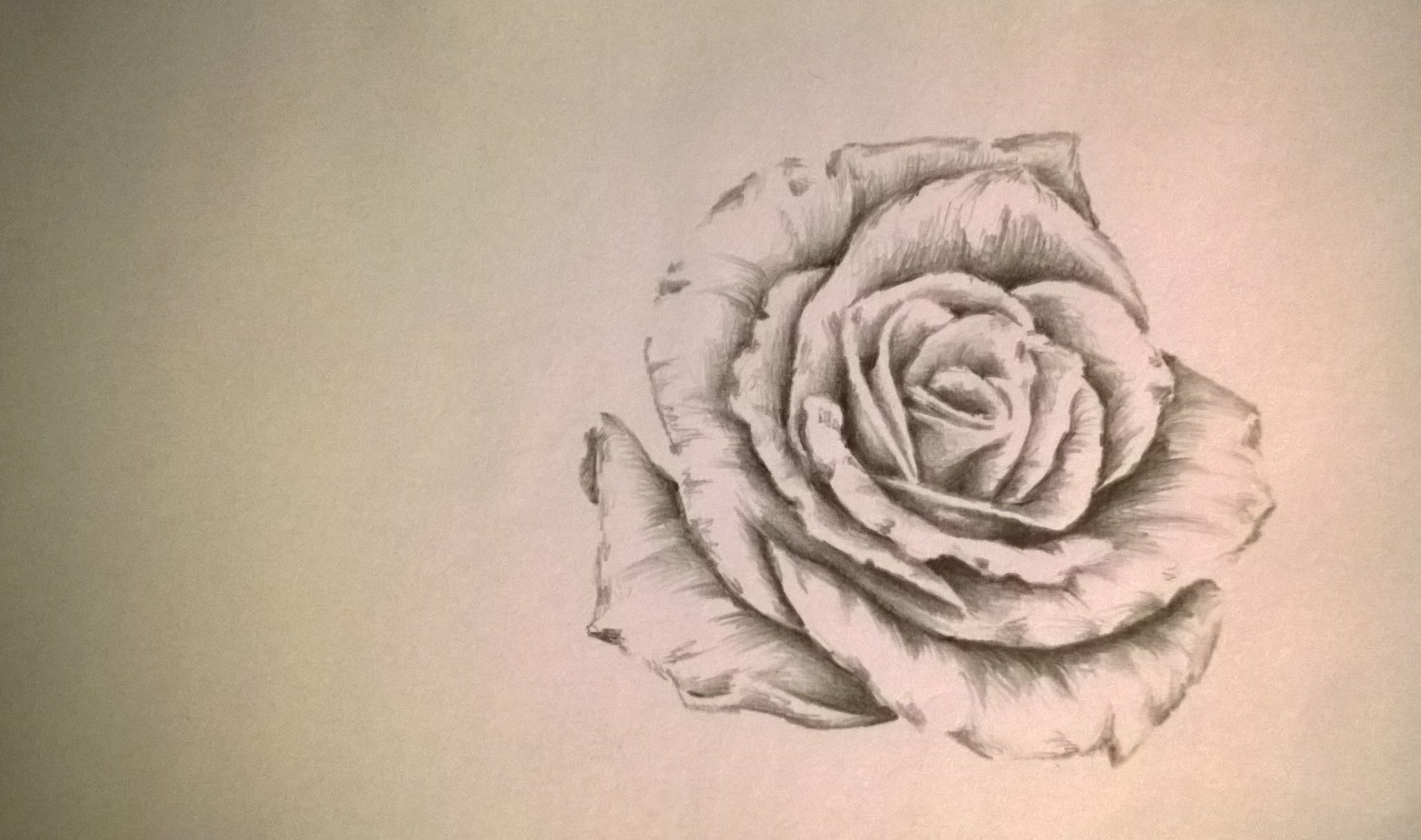The image showcases a meticulously detailed pencil drawing of a fully bloomed rose, rendered on a slightly off-white or gray sketch pad. Each petal of the rose is intricately illustrated, with the outer petals spread wide open and the inner petals becoming progressively smaller and densely packed towards the center. The high level of detail emphasizes the natural beauty and complexity of the flower. The artwork is devoid of any text, allowing the viewer to focus solely on the exquisite craftsmanship of the drawing.